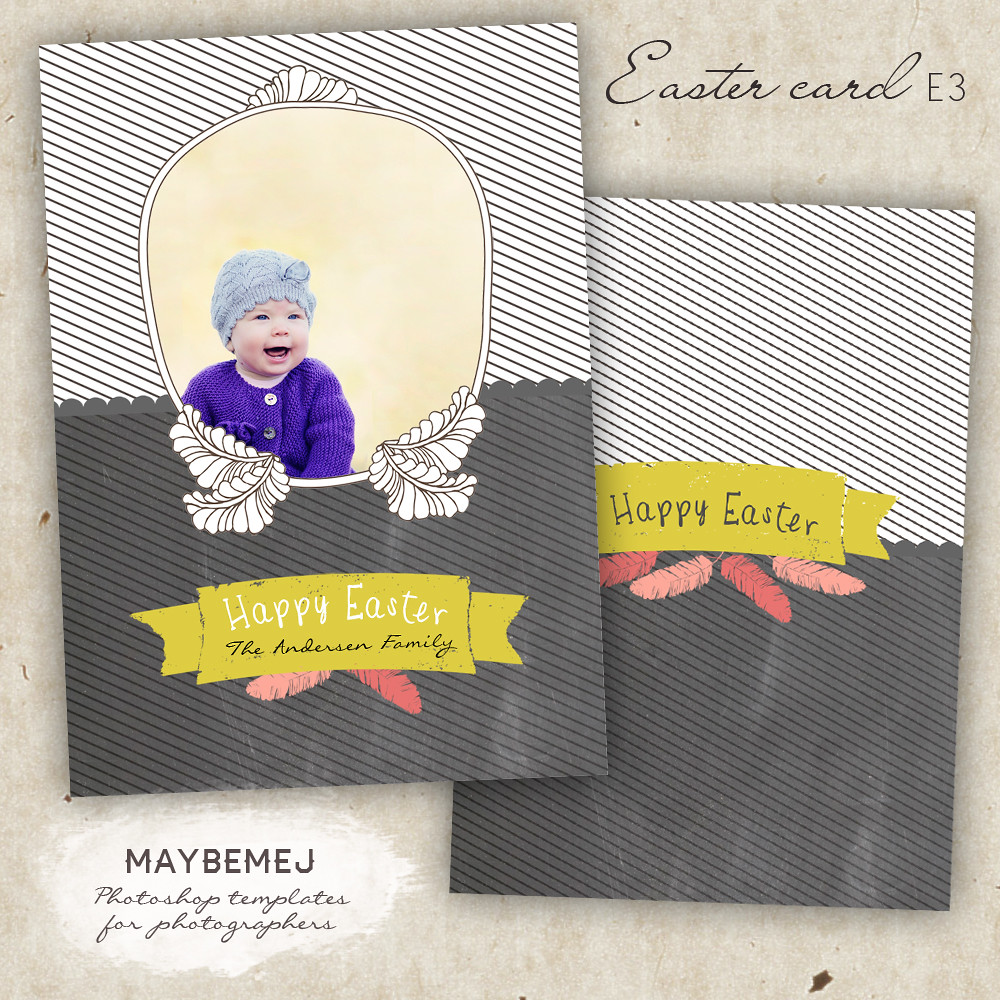This image features an Easter card template designed for photographers. The template appears to be displayed on a gray stone surface. Central to the image, two overlapping cards showcase the design from different angles. The top right of the template is labeled "Easter card E3," and the bottom left bears the text "Maybe Me Jay Photoshop Templates for Photographers."

The primary focus of the template is a black and white frame with an opening at the center, which houses a picture of a baby girl. She is adorably dressed in a purple sweater adorned with large buttons and a bluish lilac braided hat. The baby, with her blue eyes and big toothless smile, adds charm to the card. Below her photo, a yellow banner reads "Happy Easter, the Anderson family," accompanied by pink-toned feather decorations.

Behind this main template, a secondary, more simplistic card design is visible. This variant features a white-to-black gradient background from top to bottom and retains the yellow "Happy Easter" banner, along with similar feather decorations. The colors seen throughout the image include shades of tan, black, brown, light blue, purple, pink, yellow, off-yellow, red, and maroon. This image appears to be a digital advertisement for a customizable Easter card template in a Photoshop service.